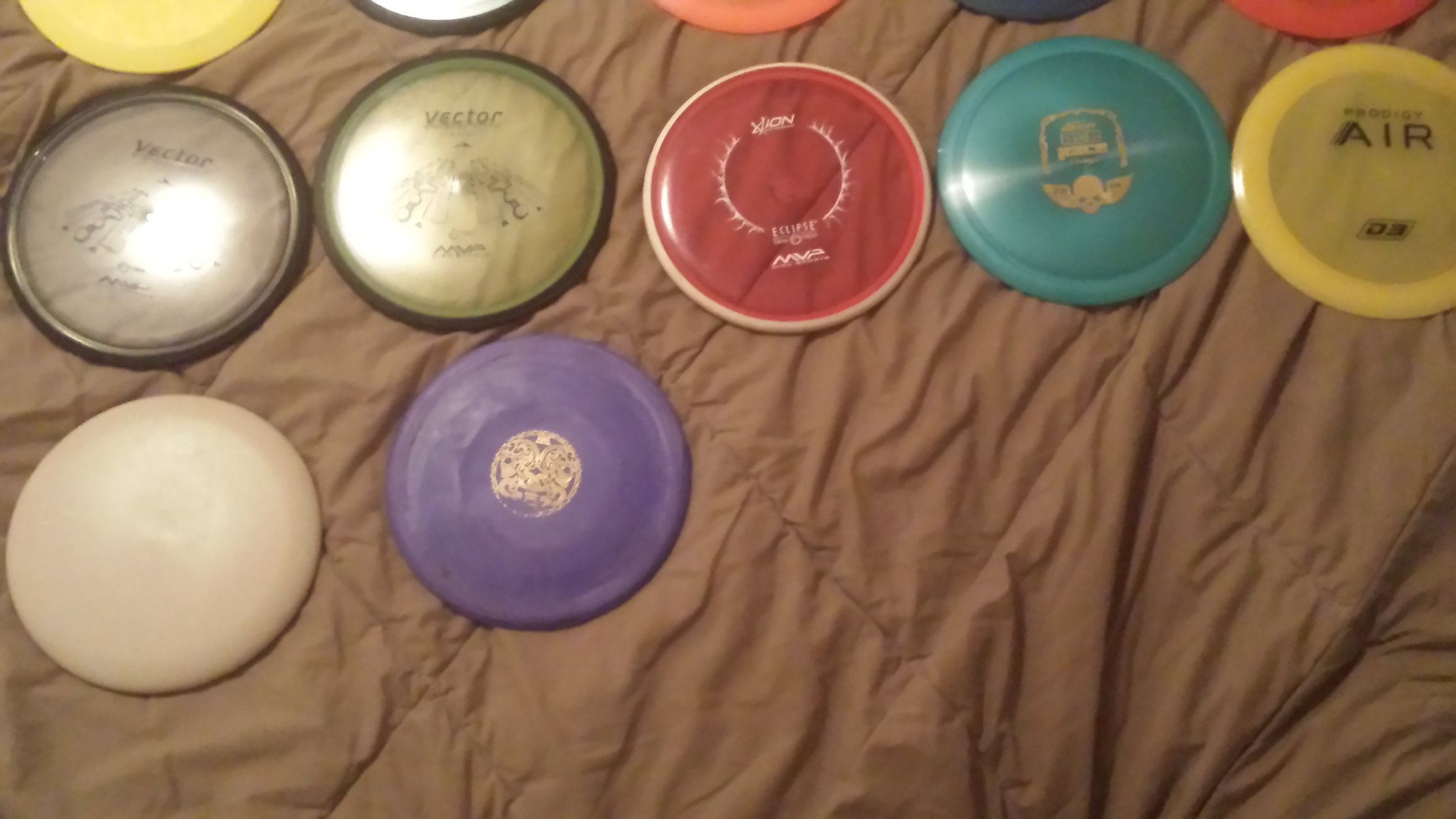The photograph captures a portion of a bed, covered with a thick, wrinkled brown bedspread, upon which a diverse collection of frisbees is neatly arranged in three rows. The uppermost row is partially visible, showing just the edges of five frisbees in various colors: yellow, white with a black outline, orange, black, and red. In the middle row, the frisbees are more distinct and possess specific designs. Starting from the left, there is a translucent silver frisbee with a black border and the word "Vector" along with an image in the center. Next to it is a green frisbee with similar features and also labeled "Vector." Following is a red frisbee adorned with sunray-like white text in the center, then a blue frisbee featuring a skull with wings design, and finally a yellow frisbee prominently displaying the word "Air" and a smaller logo beneath it. The bottom row contains just two frisbees: a plain white one and a purple one with a tiny gold logo in the center. The colorful array and varying designs suggest that these frisbees might be collectibles or part of a personal collection.